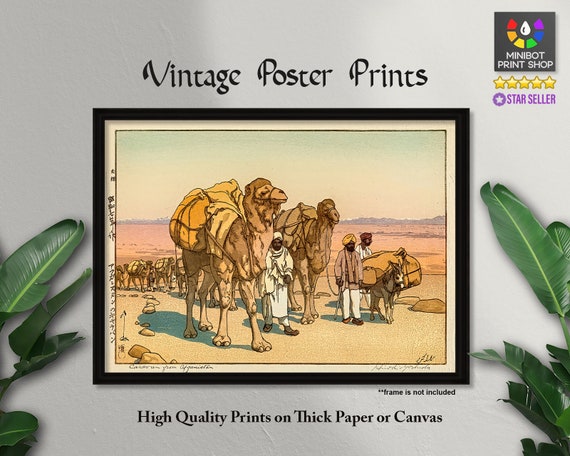The image showcases a vintage poster depicting a desert scene with camels laden with heavy loads and accompanied by three men, alongside a small donkey carrying goods. The poster is set against a grey background and bordered by green leaves on both sides. Above the image, the words "Vintage Poster Prints" are prominently displayed. The top right corner features the Minibot Print Shop logo, a white color drop surrounded by rainbow squares, followed by a five-star rating and the title "Star Seller" in purple font. The poster is promoted as "High Quality Prints on Thick Paper or Canvas" with a note at the bottom indicating that the frame is not included. This setup presents a detailed and attractive promotional display for nostalgic, high-quality prints, ideal for home decoration.